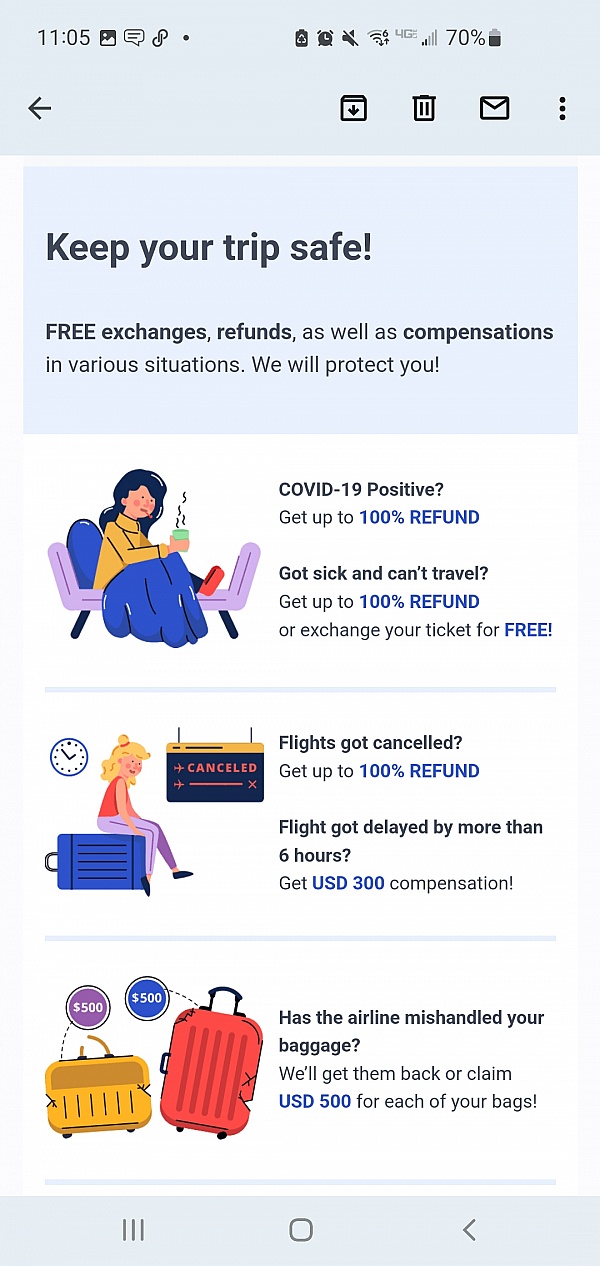Screenshot Description:
The screenshot captures a portion of a mobile phone screen with various interface elements and detailed informational text. 

In the top-left corner, the status bar has a gray background with a black time display reading "11:05." Adjacent to this, symbols appear in gray for the battery indicator, alarm clock, muted speaker, Wi-Fi with "6" next to it, "4G", and a signal strength icon showing minimal reception. A small "70%" in gray signifies the battery percentage.

Below the status bar, part of the screenshot appears to be from a photo gallery app, containing a gray and white interface. A white text box outlined by two gray lines is visible, containing ambiguous characters, including an upside-down "P" and a regular "P" in gray, and a gray circle.

More symbols follow: a gray arrow pointing left, a black-downward-pointing arrow inside a box, a black-outlined trashcan, a black-outlined envelope, and three vertical black circles.

The main content area of the screenshot transitions into a light blue background featuring a black text headline: "Keep your trip safe. Free exchanges, refunds, as well as compensations in various situations, we will protect you."

As the background turns white, detailed information about travel protection during the COVID-19 pandemic is listed:
- "COVID-19 positive, get up to," followed by "100% refund" in blue text.
- "Got sick and can't travel, get up to" followed by "100% refund" in blue text.
- "No exchange or ticket for it," followed by "free" in blue text.
- A blue line runs across the screen, indicating, "Flights got canceled, get up to," followed by "100% refund" in blue text.
- "Flights got delayed by more than six hours. Get" $300 in compensation (USD).
- "The airline is handling your baggage. We'll get them back or claim" in blue text "$500" per bag (USD).

The detailed text emphasizes various refund and compensation policies offered to travelers affected by COVID-19 and other travel disruptions.